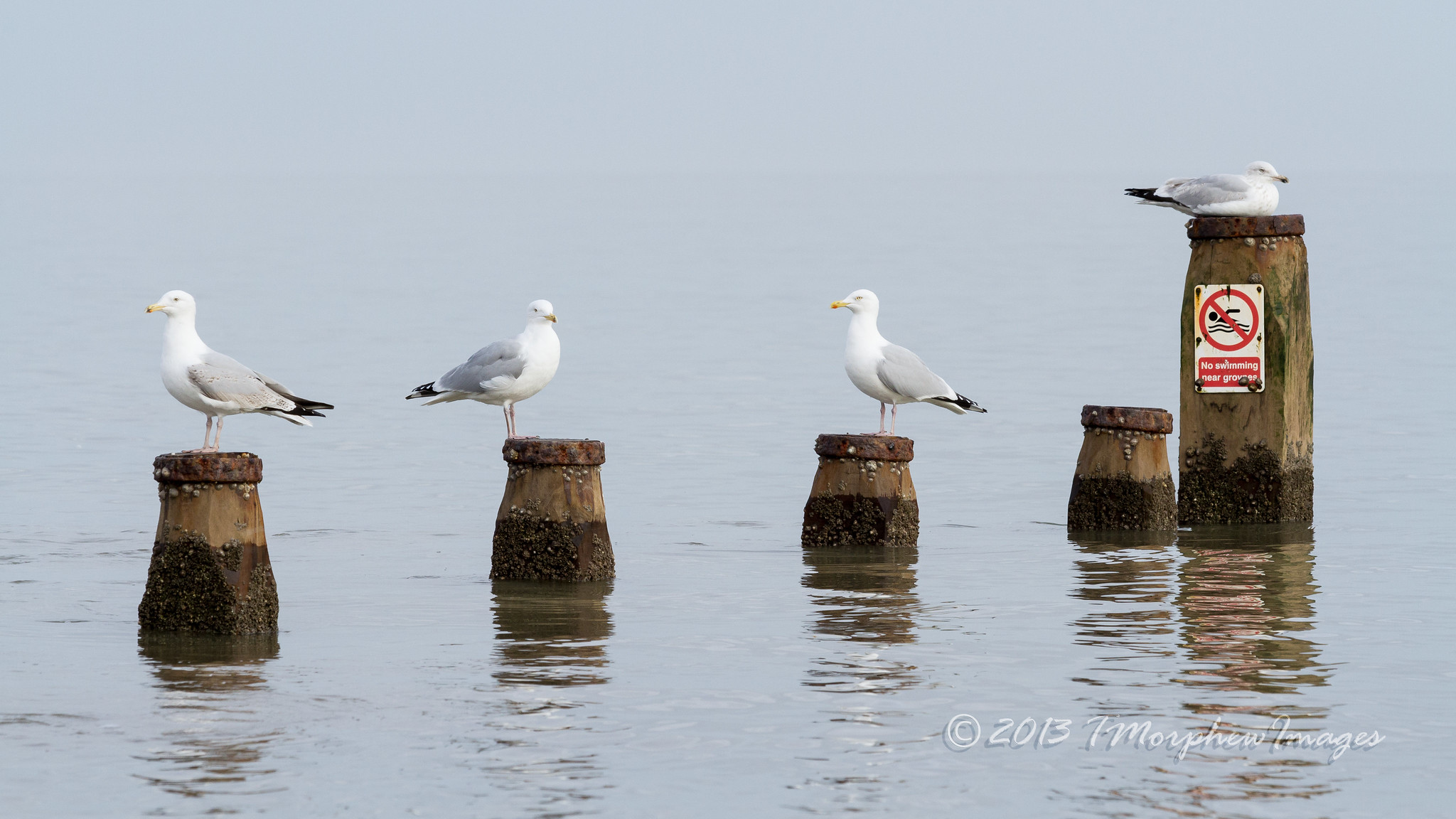The image features a serene outdoor scene with a wide expanse of gray and light blue water, merging seamlessly into a misty horizon. In the foreground, darker gray reflections and ripples shimmer on the water's surface. A line of five wooden buoys float on the water, with four of them being of uniform, shorter height, and the fifth, much taller buoy standing out at the end. This taller buoy has a white, red, and black sign nailed to it, displaying a red circle with a diagonal cross through a black silhouette of a swimmer, and below it, a red box with white text that reads, "No Swimming." Perched atop the buoys are four seagulls, white with gray wing feathers and black tail feathers, and white-yellow beaks and skinny legs. Three of these seagulls stand on their legs atop the buoys, looking in different directions, while one is seated on its belly on one of the buoys. A watermark in the bottom right-hand corner reads, "C. 2013. T. Morpheus Images."